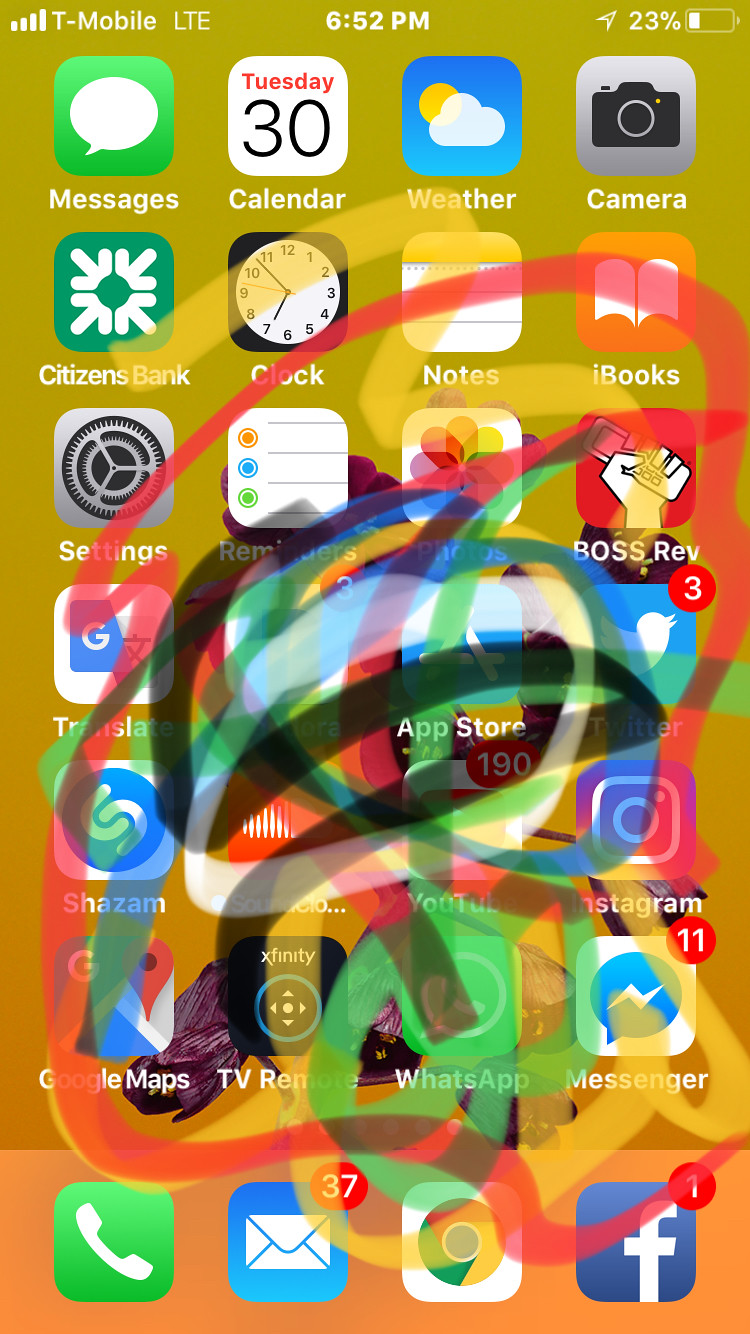This is a detailed screenshot of an iPhone's home screen, featuring a variety of popular apps against a grayish mustard yellow wallpaper. At the top, the status bar indicates the service provider as T-Mobile, with 'LTE' displayed next to it in white. The time reads 6:52 p.m., and the battery is at 23%, as shown by the battery icon in the upper right corner.

From left to right, the top row of icons includes:

1. Messages - Green and white icon.
2. Calendar - White icon with red and black detailing, displaying "Tuesday 30."
3. Weather - Blue sky with a yellow sun and a white cloud.
4. Camera - Gray background with a black camera symbol.
5. Citizens Bank - Green background featuring a white design.
6. Clock - Black background with a white clock face.
7. Notes - Yellow strip at the top, white with lines resembling lined paper.
8. iBooks - Orange background with a white open book.
9. Settings - Gray icon with a black gear.
10. Reminders - White background with an orange, blue, and green dot, lines representing lined paper.

Proceeding further:

11. Photos - Rainbow themed blossom shape.
12. Boss Rev - Red background with a white hand holding an old-style flip phone.
13. Translate - White background with a blue and gray icon; a white 'G' on the blue part.
14. An unreadable app.
15. App Store - Blue background with a white "A."
16. Twitter - Blue background with a white bird.
17. Shazam - White background with a blue circle and a white "S" in the center.
18. Another unreadable app.
19. YouTube - White background with a red square and a white play symbol.
20. Instagram - Indeterminate colors with a white camera symbol.

Continuing to the last few row:

21. Google Maps - Scribbled over, colors are unclear.
22. TV Remote - Black icon with a directional pad and "Xfinity" at the top in white.
23. WhatsApp - Green background with a white design.
24. Messenger - White background with a blue text bubble featuring a white lightning bolt inside.
25. Phone - Green icon with a white phone handle.
26. Mail - Blue background with a white envelope and a red notification circle with '37.'
27. Google (possibly) - White background, unclear colors due to scribbling.
28. Facebook - Dark blue background with a white lowercase "f," and a notification circle with '1.'

The entire screenshot is overlaid with various colorful scribbles made using the iPhone's photo editing feature, including red, green, white, and yellow marks.